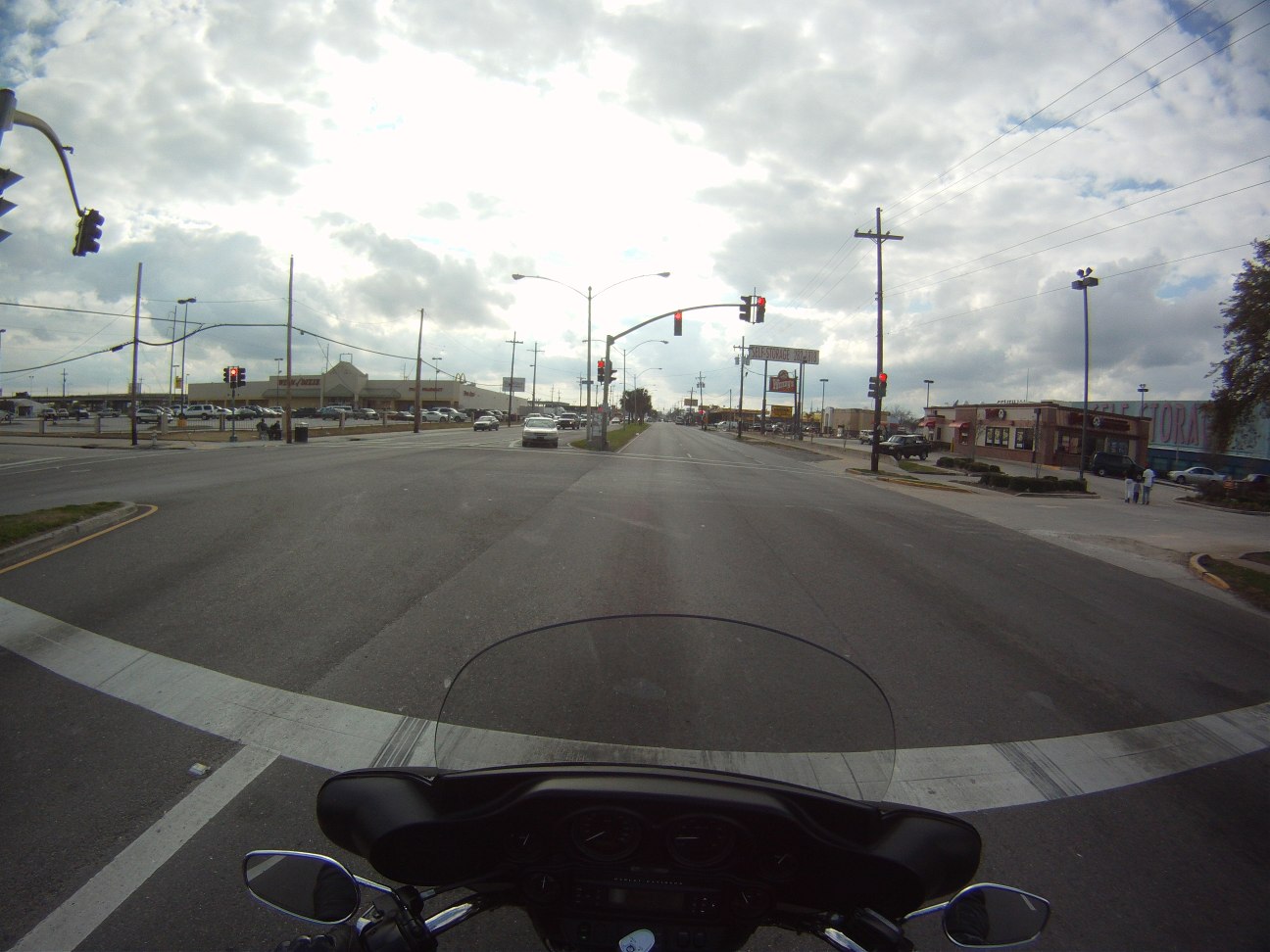The image captures an intriguing intersection from a unique perspective, likely taken from the viewpoint of someone riding a motorcycle. The scene is framed by a curved white line on the ground, which is supposed to be straight but appears distorted towards the edges, giving the impression of a wide-angle lens. On the left side of the image, there is a street light that also appears unusually curved, adding to the surreal atmosphere.

Ahead, multiple street lights show red signals, indicating a stop. At the bottom of the image, the front console area of a motorcycle is visible, complete with a small windshield and two mirrors. The street itself is gray and mostly empty, with only a few cars parked on both sides. This suggests it's a relatively quiet intersection.

In the background, on the left side, there is a large building that looks like a department store, while on the right side, a restaurant can be seen. A tree adds a touch of nature to the urban setting. The sky is filled with clouds, and a bright light is emanating from the top center of the image, creating an interesting focal point. Overall, the composition is rich in detail and offers a distinctive view of a seemingly ordinary intersection.